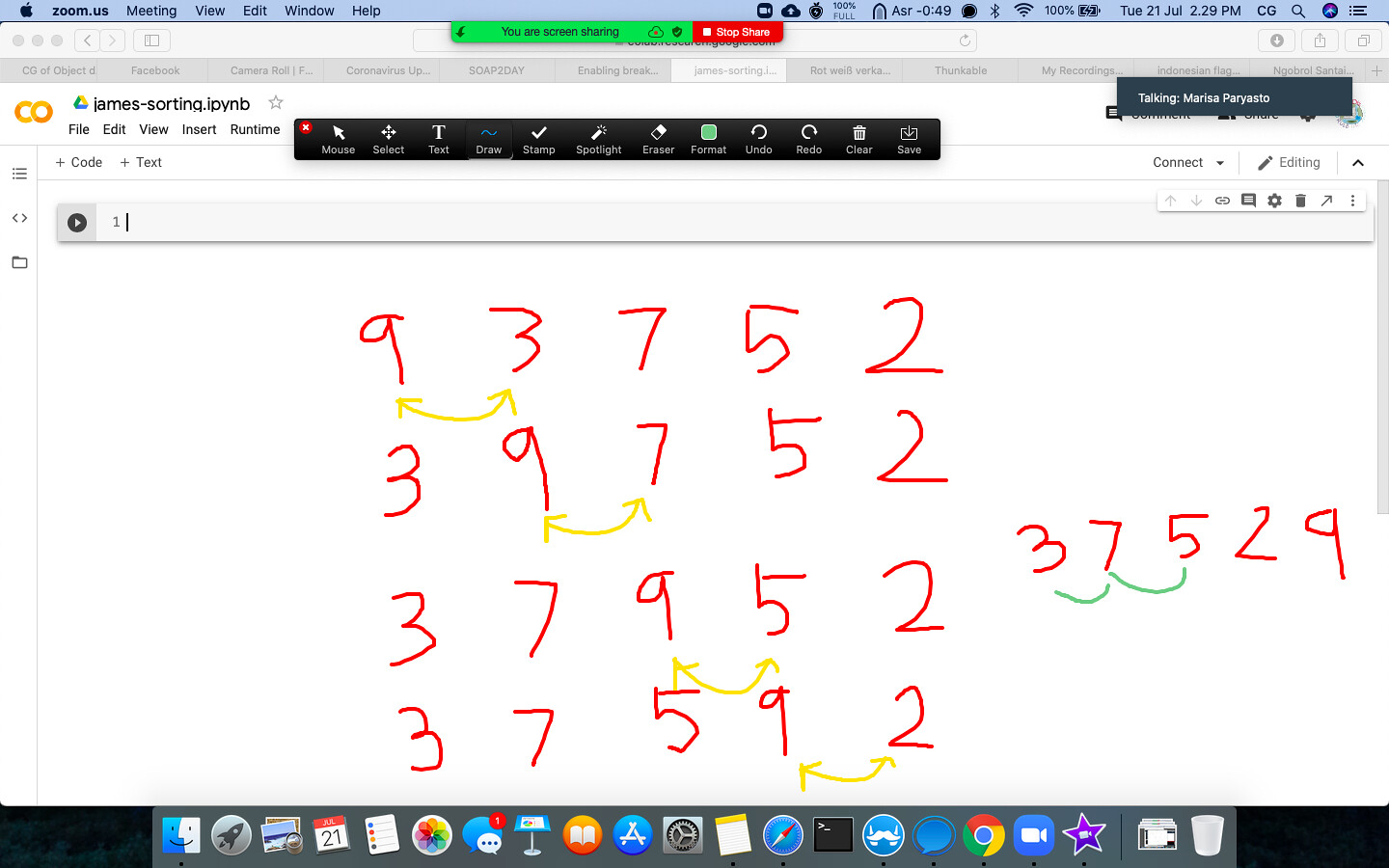The image is a screenshot of a computer screen displaying a numerical sorting process titled "James-Sorting" in the toolbar. The screen captures a sequence of number rows demonstrating step-by-step swaps to achieve a sorted arrangement. The initial top row shows the numbers 9, 3, 7, 5, and 2. 

- In this row, there is a bidirectional arrow positioned underneath the numbers 9 and 3, indicating a swap.
- In the subsequent row, after the swap, the numbers are reordered to 3, 9, 7, 5, and 2.
- This pattern continues, with each row displaying further swaps: the next row shows an arrow under the 9 and 7, and the numbers become 3, 7, 9, 5, and 2 after the swap.
- The process is repeated until four rows are displayed, each showing the intermediate steps of sorting.

To the right side of the image, the final row shows the numbers 3, 7, 5, 2, and 9. Beneath this row, two horizontal green lines span across pairs of numbers (3 and 7, 7 and 5), signifying the completion of the sorting process without further swaps. These green lines highlight the correctly positioned numbers, marking the conclusion of the sorting procedure.